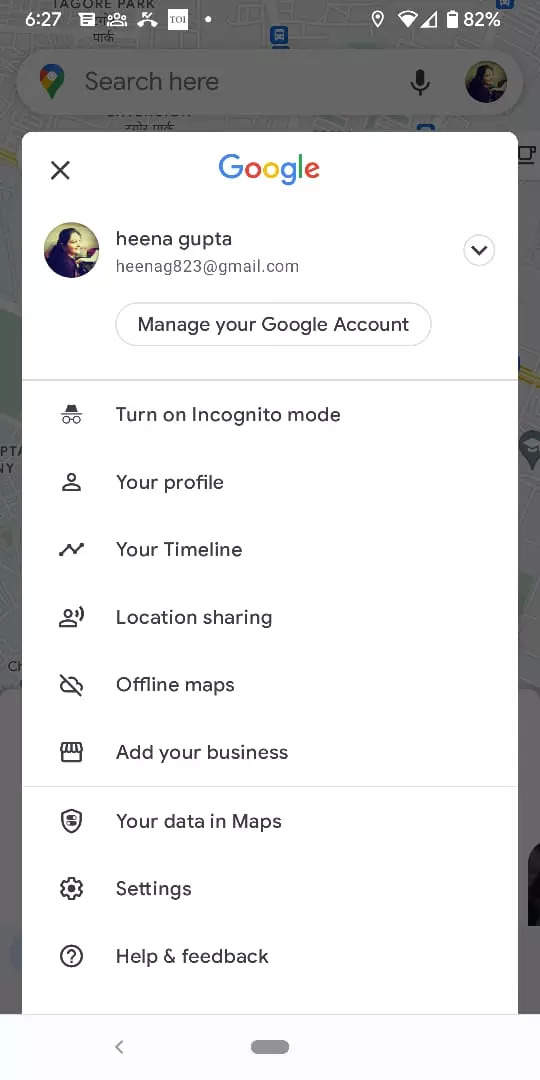This image captures a detailed view of a Google account page displayed on a smartphone. At the top of the screen, the account holder's name "Hina Gupta" is clearly visible alongside their email address "HinaG823@gmail.com." Just below this, an option labeled "Manage your Google Account" invites the user to make adjustments to their account settings.

Further down the screen, numerous options are listed. These include "Turn on incognito mode," "Your profile," "Your timeline," "Location sharing," "Offline maps," "Add your business," "Your data in Maps," "Settings," and "Help & feedback." The page background is a subdued grayish color, likely designed to minimize distractions and keep the focus on the content.

At the very top of the page, there’s a search bar labeled "Search here" and a small profile picture, presumably of Hina Gupta, echoing the user's identity and ensuring that the account details align.

The overall layout is clean and intuitive, aimed at providing quick access to various Google services and settings.